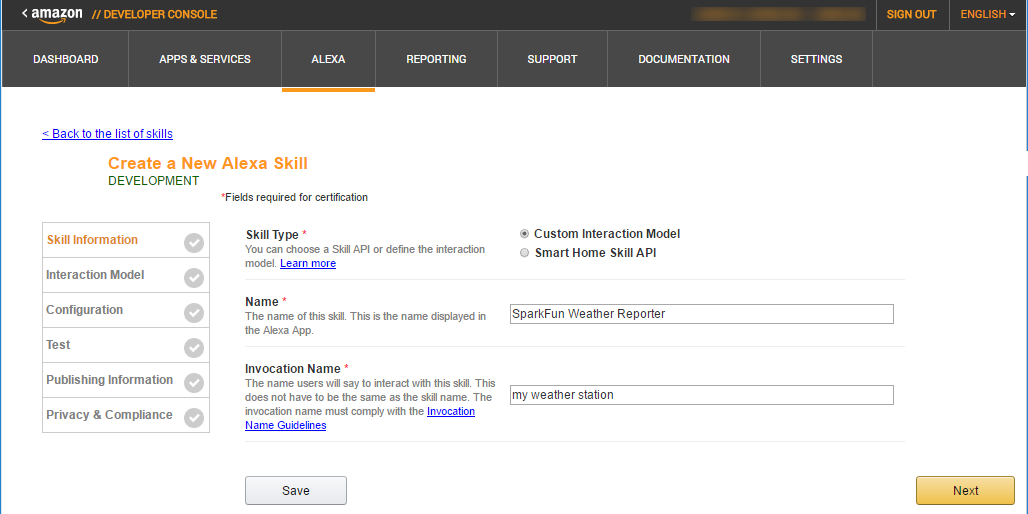The image is a screenshot of the Amazon Developer Console interface. At the top, there's a black border with the word "Amazon" in the upper left corner, followed by "Developer Console" in orange text. On the far right, there's an orange "Sign Out" button and an English language dropdown menu, all set against a gray background. 

Below this, a navigation menu composed of rectangular buttons spans the screen, including options for "Dashboard," "Apps and Services," "Alexa," "Reporting," "Support," "Documentation," and "Settings." A yellow bar beneath the "Alexa" option indicates it is currently selected. 

The main section of the screen features a white background. In the upper left corner, blue text reads "Back to the list of skills," and below that, an orange button says "Create a new Alexa skill." The word "Development" appears in green underneath.

A list of subsections runs down the left side, including "Skill Information," "Interaction Model," "Configuration," "Test," "Publishing Information," and "Privacy and Compliance," each marked with gray circles containing white check marks to their right.

On the right side, the interface shows options for "Skill Type" where users can choose between a skill API or define an interaction model. A checked circle indicates that "Custom Interaction Model" is selected. Further down, there is a field labeled "Name," where the text "SparkFun Weather Reporter" is entered. Below that, another field labeled "Invocation Name" contains the text "my weather station."

Finally, at the bottom of the screen, there is a "Save" button on the bottom left and a yellow "Next" button on the bottom right.